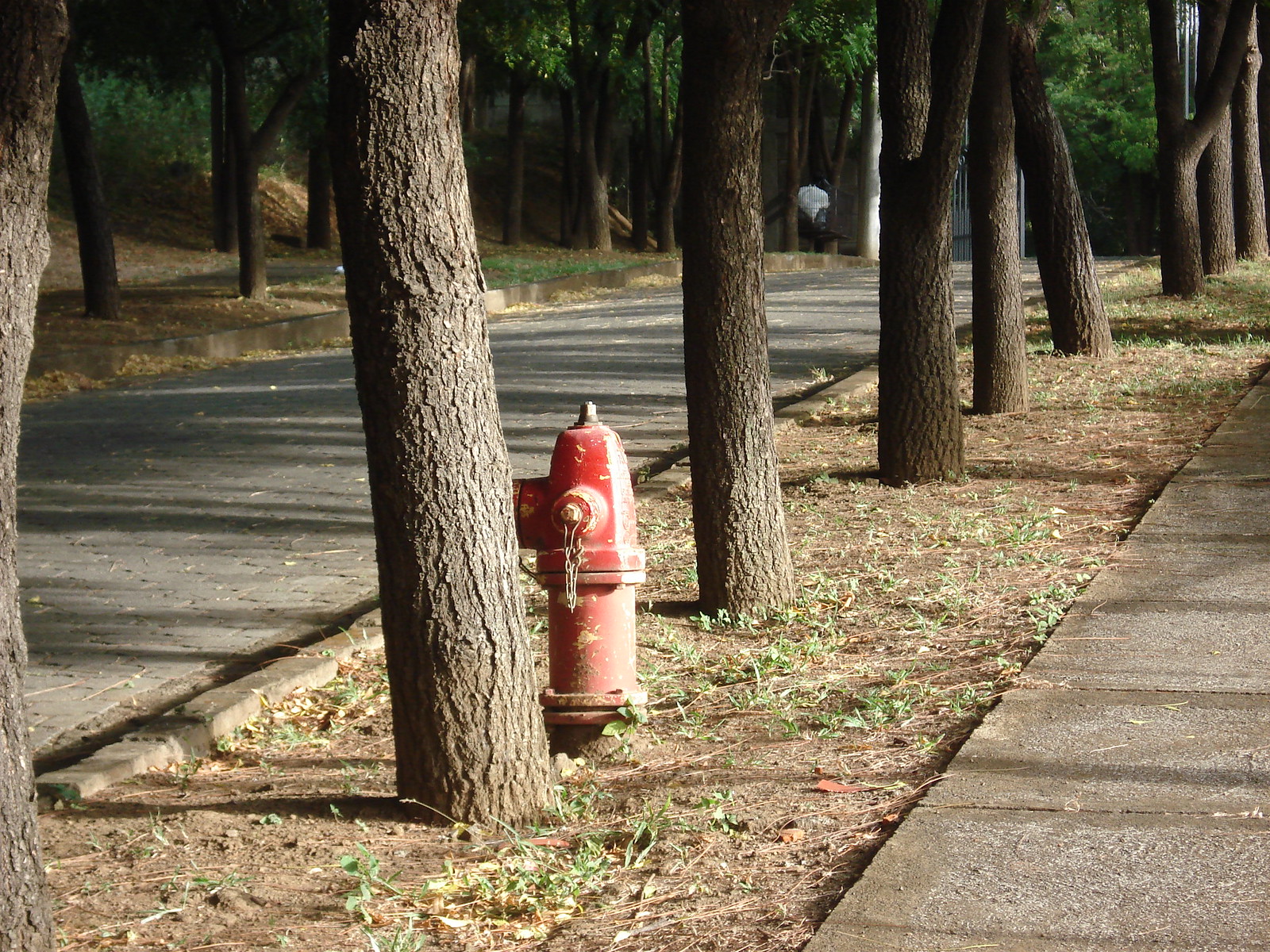This image depicts a shaded, cobblestone street lined with rows of brown tree trunks on either side. On the right side of the image, a concrete sidewalk runs parallel to the street, bordered by sporadic patches of dying grass, dirt, and scattered pine needles. Nestled between two trees, a red fire hydrant stands prominently in the foreground, featuring cylindrical extensions for hose attachment, secured by chains. Directly across the cobblestone street, further rows of trees can be seen, flanked by more dying grass and dirt. In the gutter along this side of the street, piles of fallen leaves have accumulated, adding to the scene's rustic, peaceful charm.